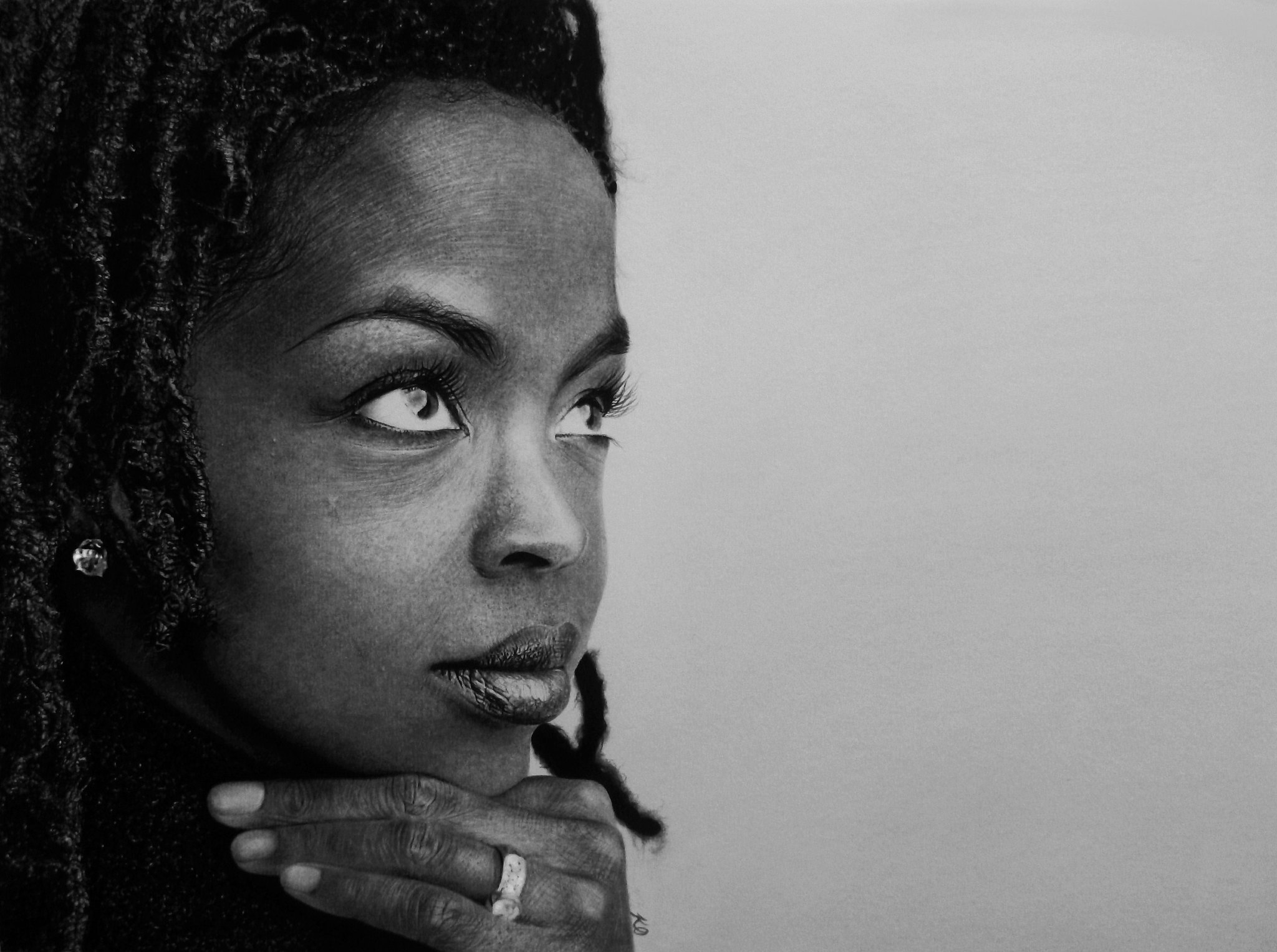A black and white photograph features a black woman positioned on the left half of the image, gazing contemplatively upwards to her left (the camera's right). She has a light gray background filling the right half of the composition. Her black hair is styled in either cornrows or dreadlocks, and she wears a diamond stud earring on her visible right ear, while her left ear remains unseen. Her left hand, adorned with an engagement or wedding ring presumably featuring a diamond, is thoughtfully resting against her chin. Her mouth is closed, and she might be wearing lipstick, although it's difficult to determine due to the monochromatic palette. Her thin fingers, trimmed eyebrows, and worn but dignified skin add to the detailed portrayal of her profile. The image, rectangular and horizontal in orientation, captures a moment of introspection in beautiful shades of gray.